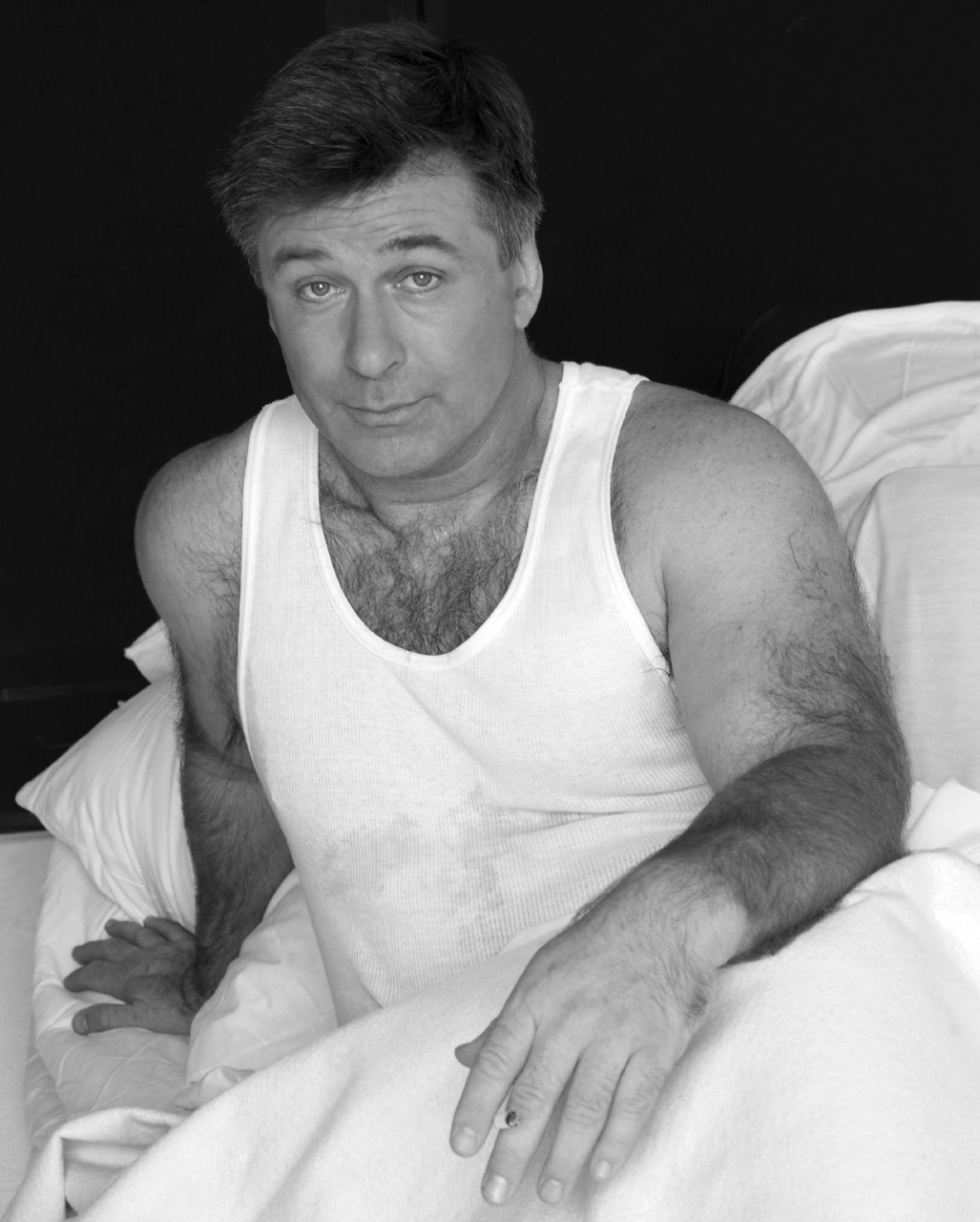The black and white photograph captures Alec Baldwin reclining in bed, surrounded by pristine white sheets and pillows against a stark black background. He is slightly propped up, supported by his right arm, and posed seductively, looking directly at the camera with raised eyebrows. Baldwin's left arm extends forward, delicately holding a cigarette between his fingers. He is dressed in a white tank top that reveals his hairy chest, arms, and forearms, and faint sweat stains are visible on his lower chest. His short dark hair and light-colored eyes contribute to the striking clarity and detail of the well-lit image.